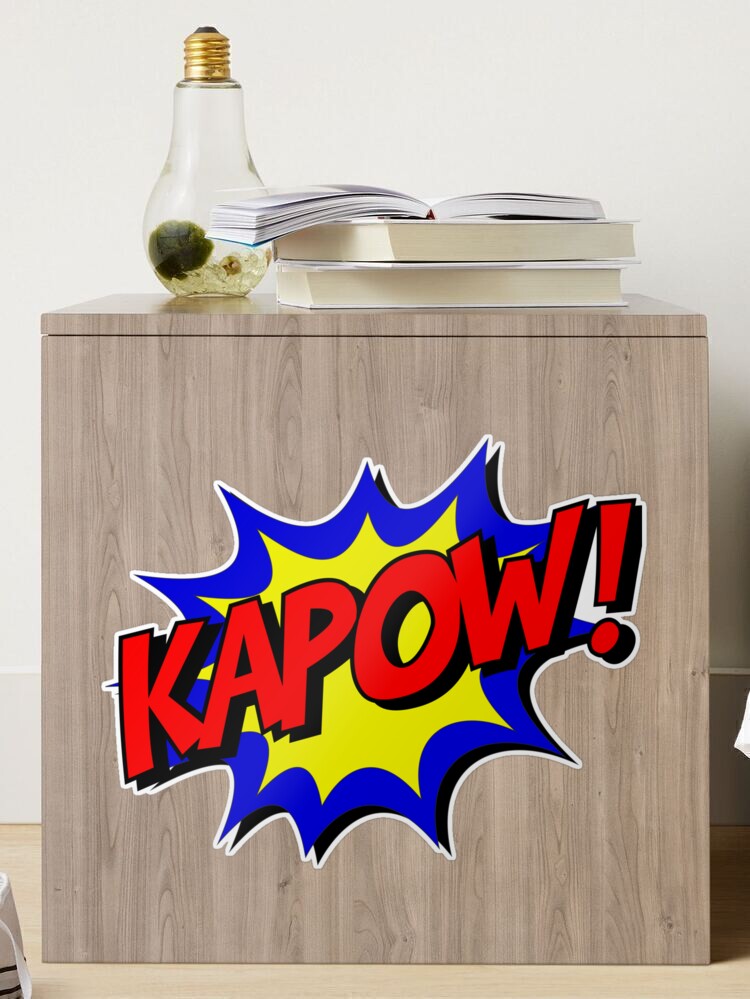This image portrays a small, wooden nightstand or side table with a distinct comic book-inspired design. The table, about two to three feet high, features a prominent "KAPOW!" text printed on its side. This text is bold and red, accompanied by an exclamation point and outlined in black, framed by a vibrant explosion effect in yellow and blue that echoes classic comic book styling.

On top of the table sit three books. Two hardcover books are stacked neatly at the base, while a third paperback book is open and placed over the stack, creating an inviting, well-read atmosphere. To the left of this book arrangement is an unusual lamp or decorative object - a clear, upside-down light bulb filled with small crystals or rocks and green moss-like details, suggesting a whimsical, perhaps nature-inspired aesthetic. The backdrop features a white wall and a light brown floor, keeping the focus on the intriguing items adorning the nightstand.